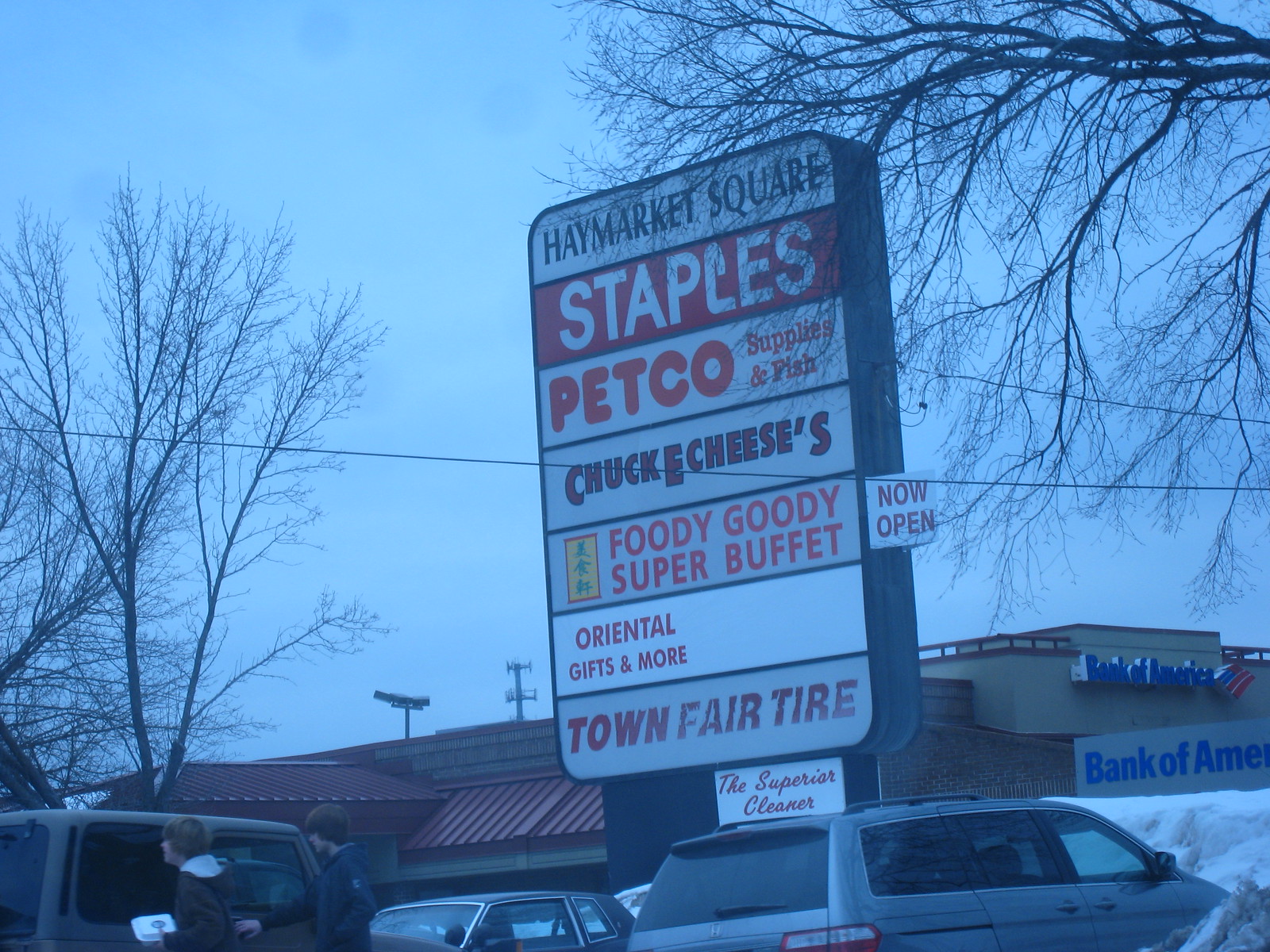The photograph appears to have a faded, bluish overlay, giving it a vintage or surreal aesthetic. The sky is a clear blue, and bare trees reach into it, intersected by prominent telephone lines. At the bottom of the image, there's a partially visible building with a few vehicles parked in front, one of which is a minivan. The building displays the Bank of America logo. 

Dominating the right side of the photo, a tall, rectangular sign lists various stores in a vertical arrangement. The sign reads as follows from top to bottom: 
1. Haymarket Square
2. Staples (with a red background)
3. Petco (supplies and fish, in red lettering)
4. Chuck E. Cheese's (in dark lettering)
5. Foodie Goodie Super Buffet
6. Oriental Gifts and More
7. Town Fair Tire
8. The Superior Cleaner

The descriptive elements capture the eclectic mix of establishments in the depicted commercial area.